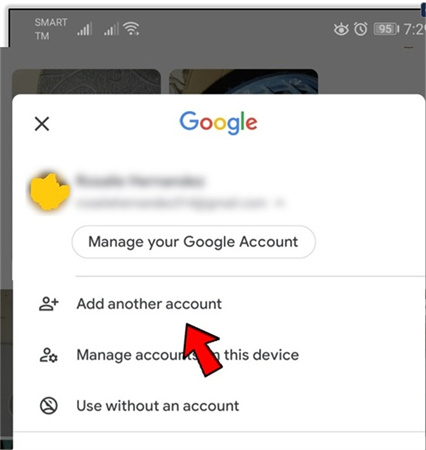In the image, we see a mobile screenshot focusing on the settings of a user's Google account. At the very top, there's a grey border, followed by the standard icons seen on a mobile device. On the far left, in small white font, it reads "SMART," with "TM" beneath it. Adjacent to this, there are two Wi-Fi signals: the first with four out of five bars filled, the second with three out of five bars filled. Next to them is another signal icon resembling an upside-down triangle with a rounded top. On the far right side, several more icons appear: an eye-like icon with three 'eyelashes,' an alarm clock, a nearly full sideways battery icon showing "95" in white, and the time '7:20.' However, the rest of the time is cut off.

Beneath these icons, a background with partially visible rectangular images is occluded by a prominent white pop-up window, a typical feature seen after engaging with Google settings. This pop-up features a black X in the top left corner, and in the center, the Google logo in its distinct colors. Below, where a user's avatar, name, and email would normally appear, the avatar is obscured by a yellow, blob-like scribble made in MS Paint, and both the name and email are blurred out.

The pop-up contains a button labeled "Manage your Google account," followed by a thin grey separator line that extends nearly the full width of the pop-up. Below this line, three options are listed: "Add another account" with an icon resembling a profile picture and a plus sign, "Manage accounts on this device" with a profile picture and a settings icon, and "Use without an account" featuring a profile picture with a line through it. The section concludes with a thin horizontal line spanning from left to right.